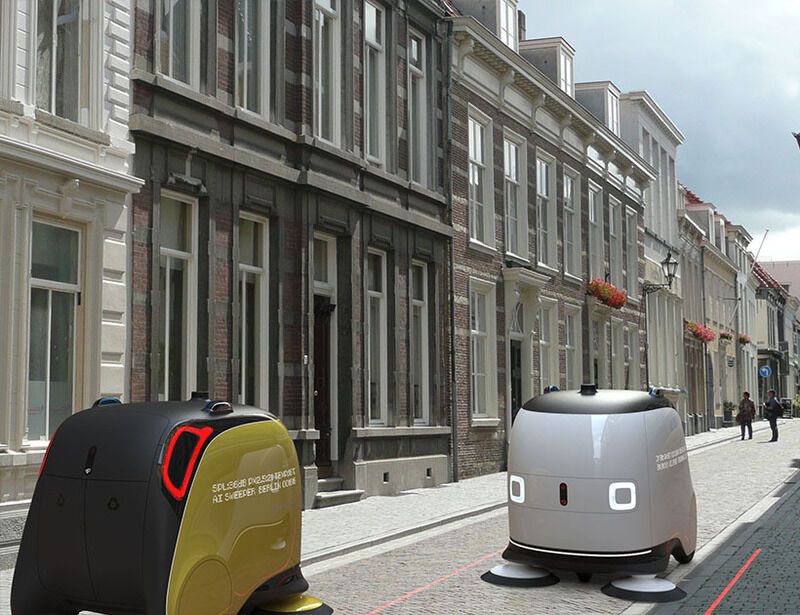The image appears to be a digitally enhanced rendering of a quaint European residential street, characterized by its tightly packed, two to three-story buildings painted in shades of white, light gray, and dark gray. These homes, aligned in a neat row, feature several windows on their facades. Along the street, near the bottom of the photograph, two robots can be seen moving in a sequence. The leading robot, designed with a predominantly black and gold body adorned with red lights along its sides, appears to be a sophisticated machine. Following closely behind is a second robot with a black and silver exterior, equipped with prominent white rectangular eyes and featuring rotating brush elements suggestively used for street sweeping. Notably, it has a single wheel at the back. Additional digital text overlays on the image read "AI sweeper" alongside other white inscriptions, indicating the robots' intended functions, thereby suggesting this image may have been edited to showcase futuristic street-cleaning technology.